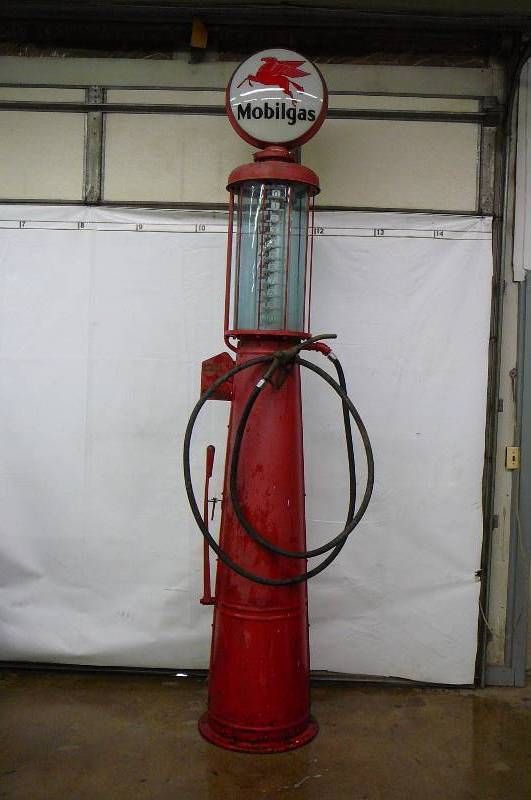In this detailed photograph, there is a striking, antique gas pump from Mobil Gas prominently featured. The tall, red pump showcases the iconic Mobil Gas logo with the winged red horse, Pegasus, set against a circular light at the very top, highlighting the brand name beneath. The pump's structure is predominantly cylindrical, widening towards the bottom where it forms a conical base. The glass-tinted cylinder in the center, enclosed by metallic bars, once served to display the amount of gasoline being dispensed. This nostalgic artifact, appearing to hail from the 1950s, stands in a garage with a glossy brown floor, against what seems to be a white garage door. The black hoses hang centrally from the pump, adding to its vintage charm, while the nozzle shows signs of rust, indicating years of disuse. This evocative image captures not just an old gas pump, but a piece of automotive history preserved in a private garage.